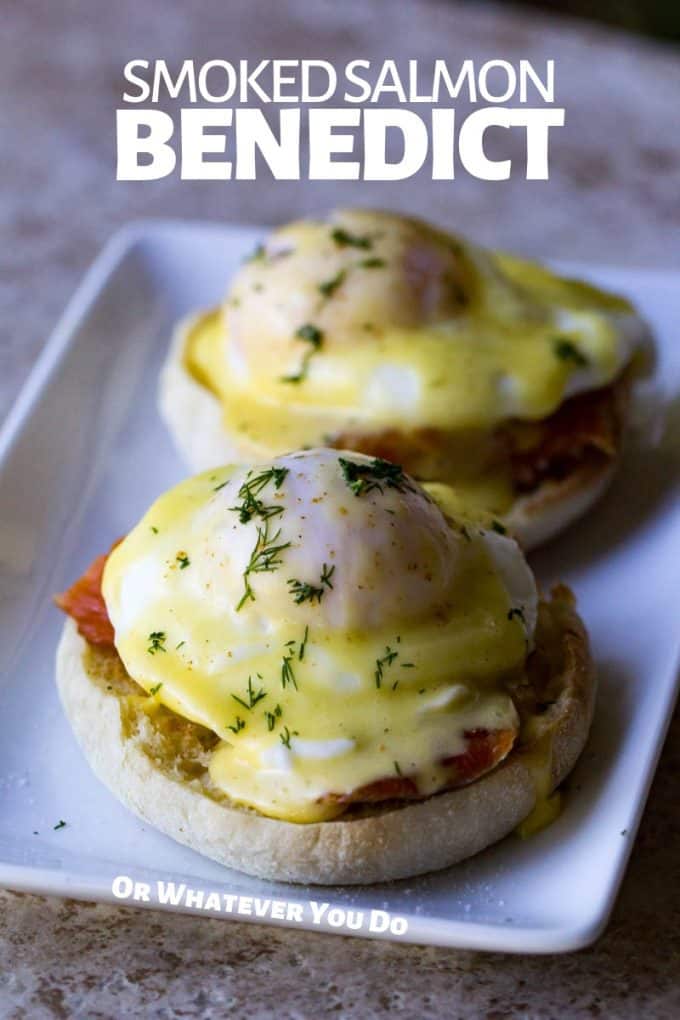The image is an extremely close-up photograph of an eggs benedict dish on a white, raised, edged ceramic plate. The plate is diagonally oriented and sits on a multicolored, textured countertop, possibly marble, suggesting it could be in a kitchen or a restaurant. The dish features two vertically-aligned English muffin halves topped with smoked salmon, and an eggs benedict, characterized by a white and yellow mixture from the hollandaise sauce and egg yolk, adorned with a green garnish resembling rosemary. The image's text elements include the phrase "smoked salmon Benedict" in thicker, bolder white text at the top, while at the bottom edge of the ceramic plate, it reads "or whatever you do." The overall scene is well-lit, emphasizing the dish's vibrant colors, including shades of brown, white, yellow, and orange.